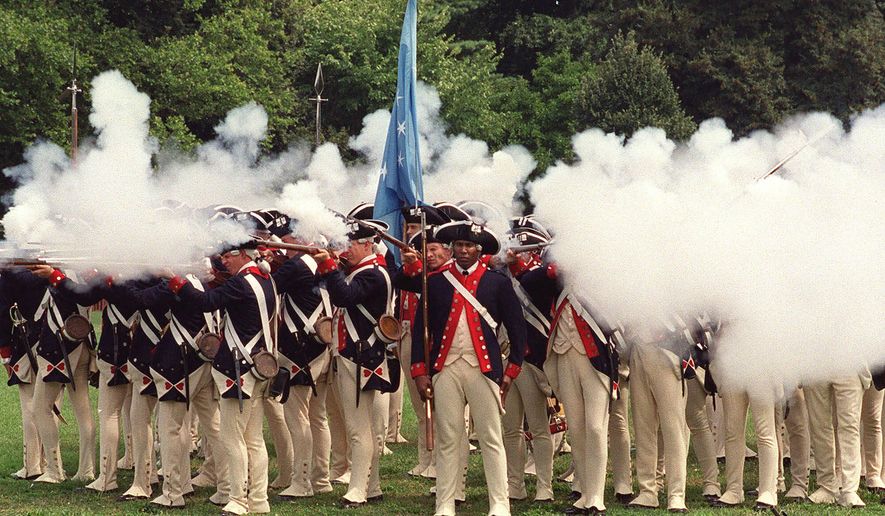In this vibrant, clear outdoor photograph taken in landscape orientation, a group of men are participating in a Revolutionary War reenactment. Each man is adorned in period-specific attire, featuring white, cream-colored trousers, and navy blue jackets with red lapels and brass buttons. They complete their historic look with dark blue, triangular felt hats trimmed with white at the edges and white wigs. The men are arranged in several rows, primarily aiming and firing large muskets to the left side of the composition, resulting in visible clouds of white gun smoke.

The setting is lush, with dark green trees forming a natural backdrop and grass beneath the men’s feet, all bathed in bright, clear daylight. Central to the scene, a man is prominently holding an American flag on a pole, facing the viewer amid the surrounding smoke. His distinct position and lack of smoke enveloping him make him a focal point. The overall impression showcases representational realism, capturing the essence of a lively historical reenactment rather than an antique war scene, underscored by the photograph's modern clarity and vibrancy.